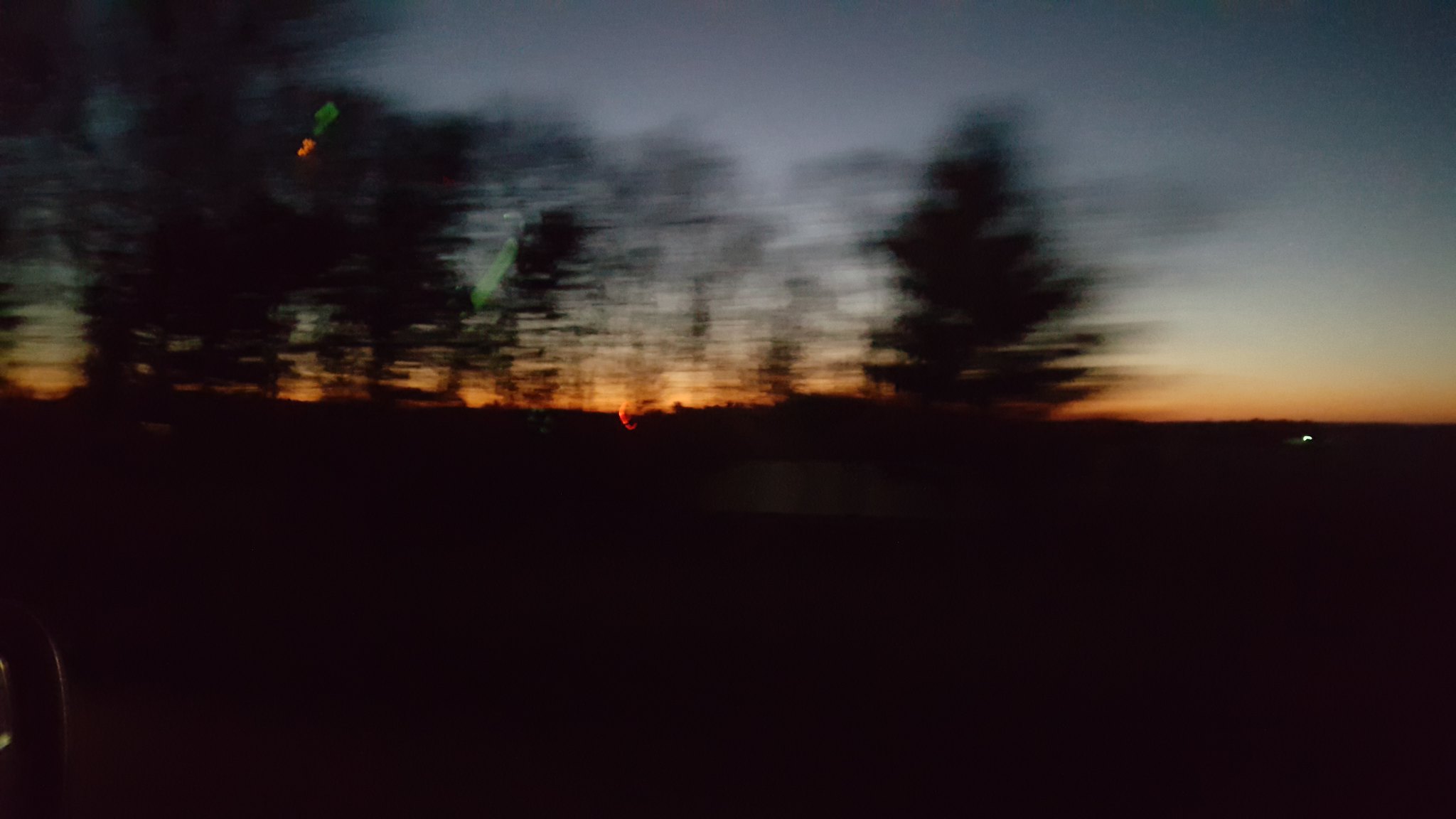A blurry photograph captures a dynamic, almost surreal scene with various elements beautifully framed. The image features a mixture of blurred trees, some dense with foliage and others bare, emphasizing their distinct forms. There is a prominent green streak running between some trees, juxtaposed with orange and green light distortions that add an abstract quality to the image. A soft white flare further diffuses the scene. The photograph appears to have been taken from a moving vehicle, hinted at by the outline of a car mirror visible on one side. In the sky, a gradient from orange to blue and white suggests either dawn or dusk, with darkening hues above adding depth. In the distant background, there is a faint, blurry light on a building, contributing to the overall dreamy, ethereal quality of the photograph.